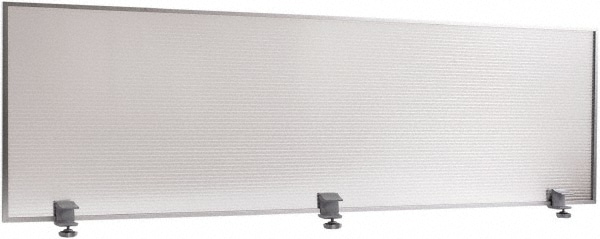The image depicts a narrow, long rectangular screen or panel, resembling a desk or cubicle divider, characterized by a light silver or grayish hue. The surface of the panel is detailed with small horizontal ridges running along its length. Encasing the panel is a thin, dark gray frame that transitions to a lighter color at the bottom, with the entire structure slightly slanted, making the right side appear further and lighter, as though illuminated by sunlight. At the bottom edge of the panel, there are three pieces of hardware or attachments: one on each end and one in the middle. These attachments serve to secure the panel to a surface, likely a desk, with mechanisms that appear to tighten for stability. The overall composition suggests a functional piece of office furniture designed to provide privacy or separation.